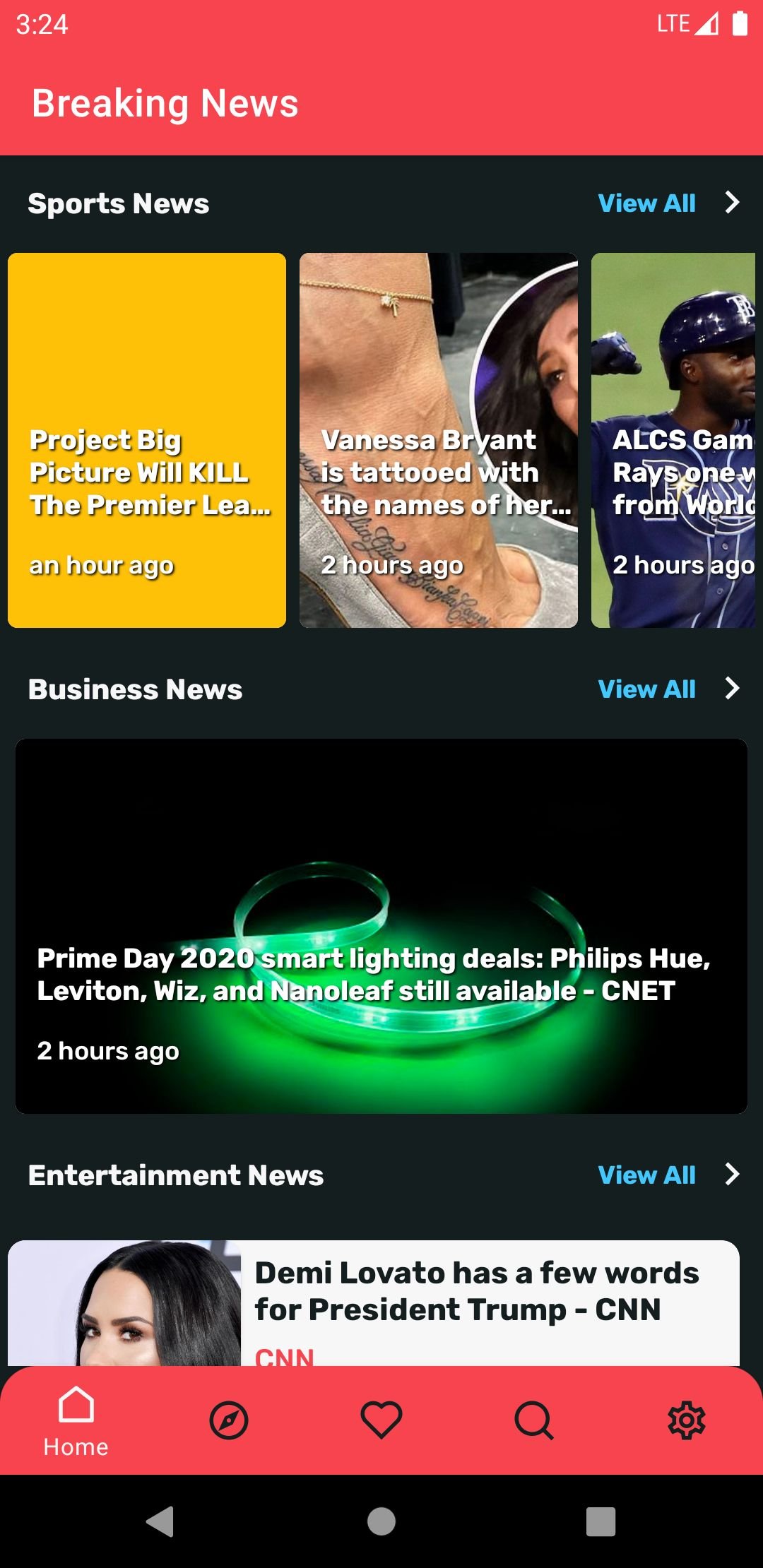This is a screenshot of a smartphone displaying a news feed with various sections. The top part features a status bar within a red box, showing the time "3:24," full battery life, and strong signal strength. Below, in bold red text, it reads "Breaking News."

The background of the news feed is black. The first section is labeled "Sports News," with an option to "View All" on the right. The headline reads, "Project Big Picture will kill the Premier League," marked as posted an hour ago. Following this, there's another headline, "Vanessa Bryant is tattooed with the names of her...", which seems incomplete.

Further down, under the section titled "Business News," there’s a headline about Prime Day deals: "Prime Day 2020: Spotlighting Deals – Philips Hue, Leviton, Wiz, and Nanoleaf still available on CNET," posted two hours ago.

Next is the "Entertainment News" section, with an option to "View All" in blue on the right. The headline here states, "Demi Lovato has a few words for President Trump," attributed to CNN.

At the bottom, there's a navigation bar with red icons for Home, a Steering Wheel, a Heart, a Search symbol, and Settings. Beneath this is another black bar featuring buttons for Home, Back (an arrow), and Close (a square).

This detailed caption describes the layout and contents of the screenshot, providing insight into the type of news displayed and the functionality of the navigation bars.